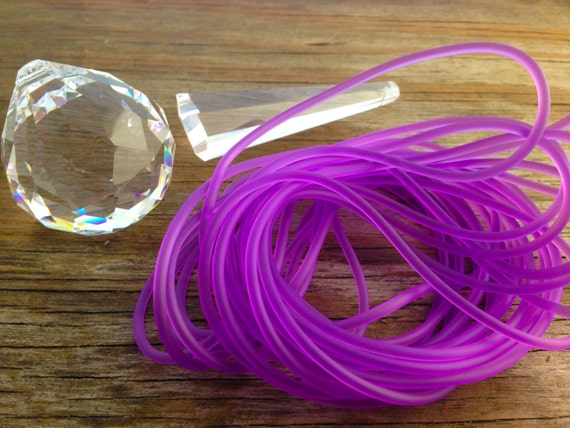This photograph, taken from an overhead perspective, captures a weathered wood table of browns and grays adorned with three distinct objects. To the top left, a multi-faceted, clear crystal globe refracts an array of colors—purple, turquoise blue, yellow, and white—creating a vibrant prism effect. Adjacent to it on the right lies a sphere-like crystal with one end tapering into a nipple-like point, also dispersing a spectrum of colors. Below these crystals rests a large loop of translucent, flexible neon purple nylon cord, appearing akin to a wound-up fishing line or jump rope, adding a vibrant, electric touch to the composition.